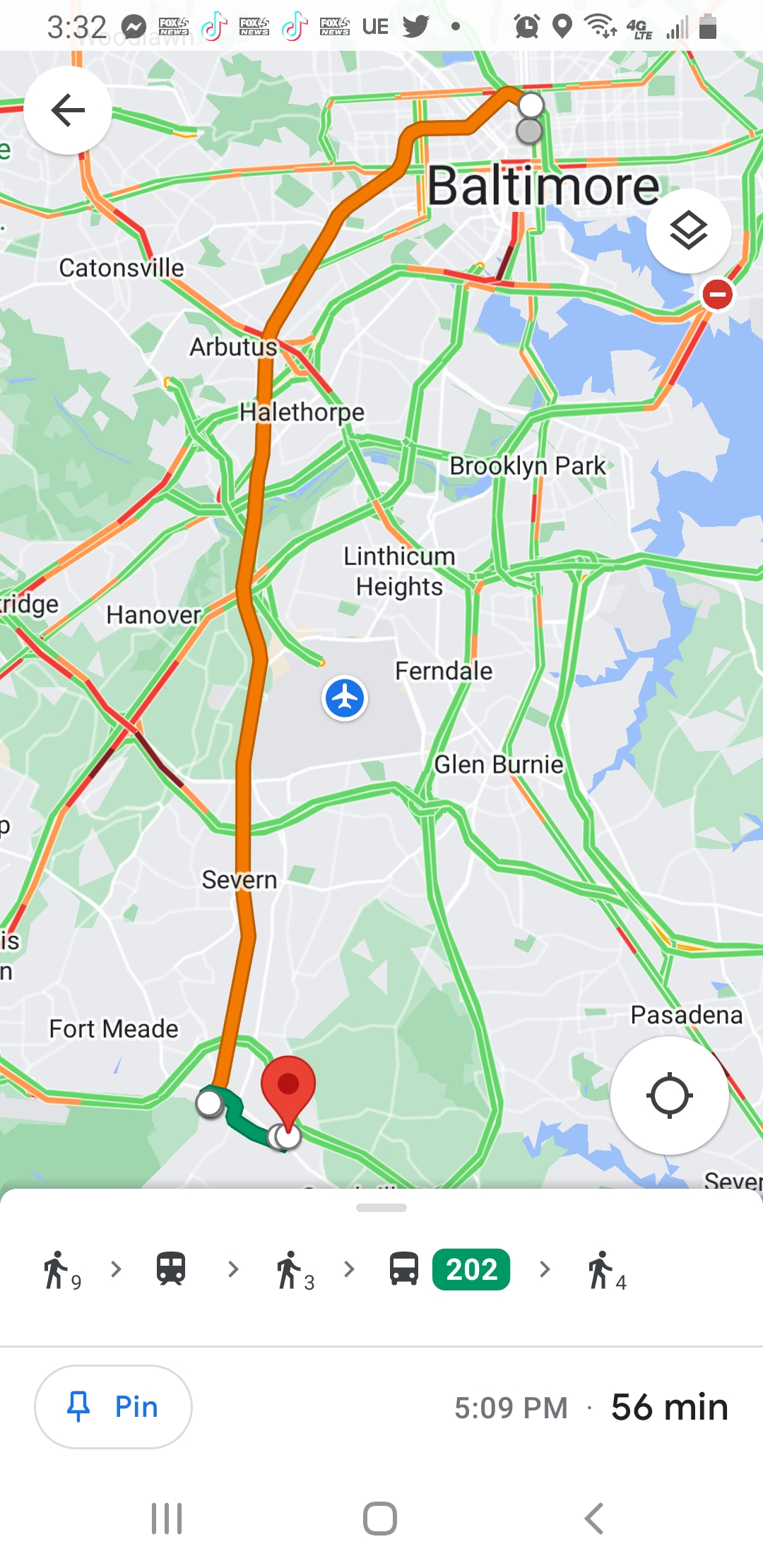The image depicts a smartphone screen showcasing a map interface prominently in the center. The map is crisscrossed with various lines in multiple colors—white, red, green, and orange—likely representing different routes or traffic information. At the bottom of the screen, there are three distinct icons arranged from left to right: the first icon features three vertical lines, the second icon is a simple square, and the third is a directional arrow pointing left. Above these icons, there is a blue location pin marked with the word "PIN" to its right. Adjacent to this label is the number "5", providing further context, possibly indicating a location marker or a numerical reference on the map.